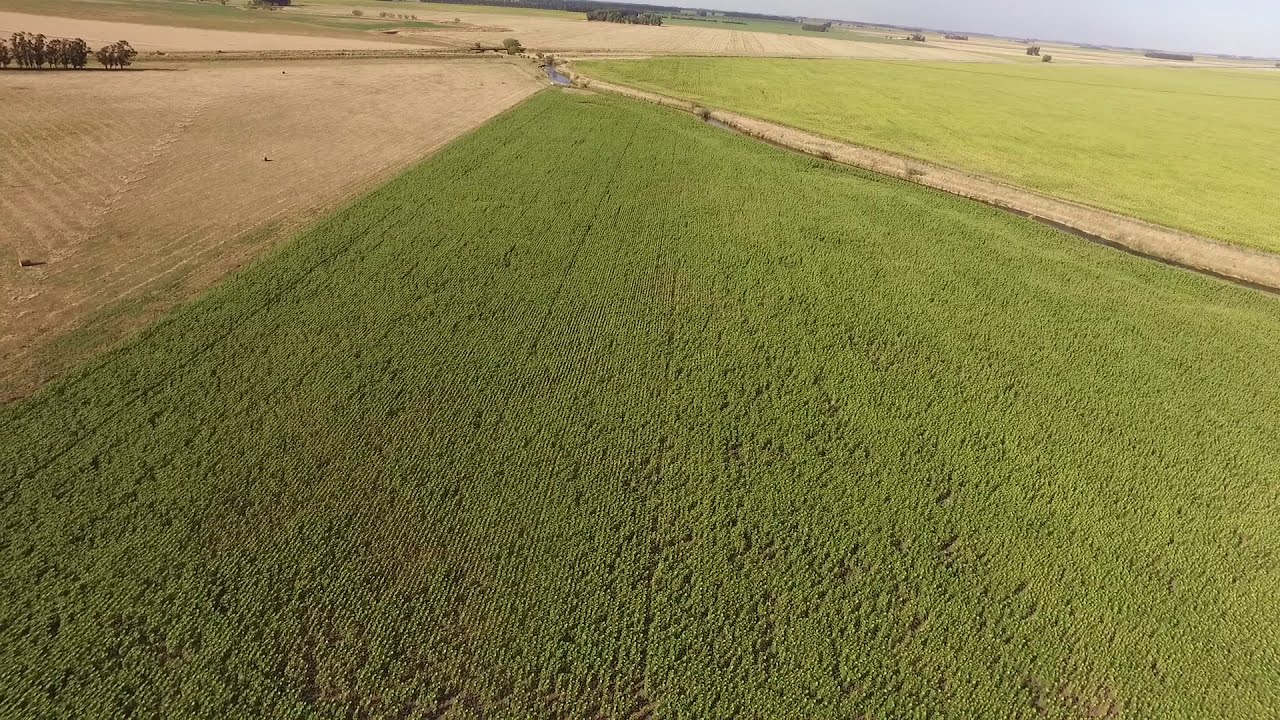The image is an aerial photograph capturing a vast, open farmland landscape during the middle of the day on a cloudy day. The scene predominantly features a mosaic of green and tan fields, spread out in an orderly, well-spaced manner across the frame. The fields are divided by a dirt road that starts from the middle right and extends diagonally to the top left, where it splits. A distinct dividing line runs from the top left to the top right, segmenting the fields into different sections. On the left side of the dividing line, there is a large expanse of green fields mixed with some areas of dirt, while on the right side, the green fields are denser with neatly planted rows of crops.

In the top left corner, the fields transition to a tan color, likely indicating either a wheat field or a plowed area. Sparse grass fills the spaces between these sections. The road running through the image features fields of grass on both sides up to the upper right corner, with more greenery extending beyond it. Scattered trees and farmhouses can be seen on the far right, along with a touch of light blue sky in the upper right corner, adding to the image's expansive, serene rural atmosphere. No text or additional markings are present within the image.